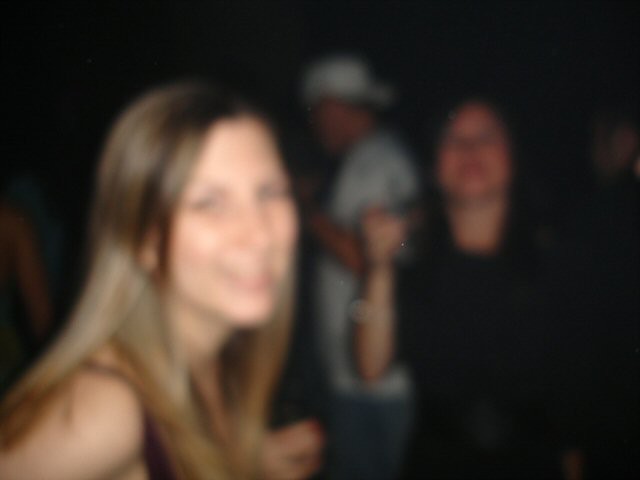In this somewhat blurred, dimly lit photograph, three people can be seen amidst what appears to be a gathering or nighttime event. The woman closest to the camera, a Caucasian with long blonde hair and blue eyes, beams a wide smile while wearing what seems to be a strapless top or a tank top with a black strap visible over her shoulder. To her right and slightly in the background, another woman, possibly white or Hispanic with dark hair, dons a black shirt or dress. Her face has a reddish hue and she is gesturing towards the camera with her right arm raised at the elbow, her chin lifted upwards. At the very back, a man wearing a white t-shirt, blue jeans, and a backwards baseball cap faces away from the camera, blending into the darker areas of the image. Despite the blur, the scene captures a lively moment, possibly with dancing, among the trio.